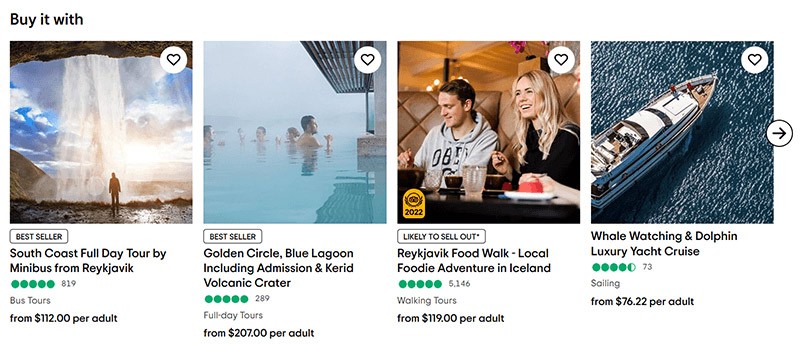The image is a collage of four travel options, designed to captivate potential tourists with picturesque and enticing experiences. Each segment showcases a different tour, complete with ratings, reviews, and pricing.

1. The first segment features an adventurer standing under a rocky overhang, adjacent to a majestic waterfall cascading under a clear blue sky. The caption informs us it's a "Best Seller" tour: the "South Coast Full Day Tour by Minibus from Reykjavik." This highly-rated excursion boasts five stars from 819 reviews and is priced from $112 per adult.

2. The second section highlights another "Best Seller," depicting men and women enjoying a refreshing dip in the water with a dock visible in the background. This segment advertises the "Golden Circle, Blue Lagoon, including admission, and Kerid Volcanic Crater" tour. Garnering five stars from 289 reviews, this full-day tour starts at $207 per adult.

3. The third portion, labeled "Likely to Sell Out," presents a vibrant scene of two people laughing and enjoying a meal at a bar or restaurant. It promotes the "Reykjavik Food Walk Local Foodie Adventure in Iceland," a gastronomic journey that has earned five stars from an impressive 5,146 reviews. Walking tours for this delightful experience begin at $119 per adult.

4. The final section captures a luxurious yacht sailing on the ocean, promising an idyllic whale-watching and dolphin-spotting escapade. This tour, titled "Whale Watching and Dolphin Luxury Yacht Cruise," has received four and a half stars from 73 reviews and is available from $76.22 per adult.

Together, these images compile a diverse array of top-rated travel experiences, each offering a unique way to explore and enjoy the rich landscapes and culture of their respective regions.